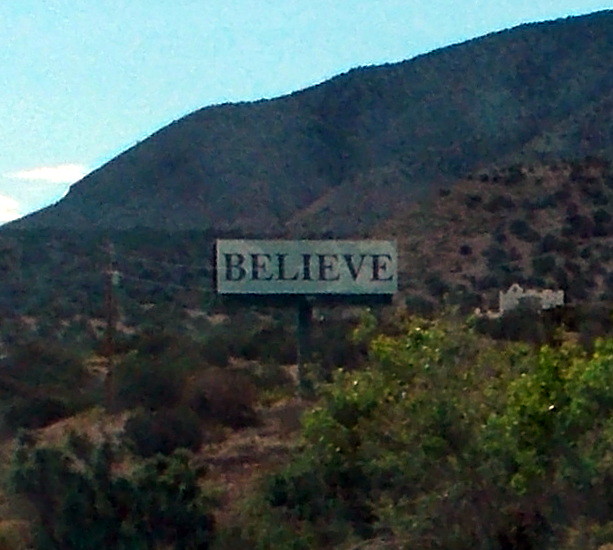In this rather low-resolution photograph of a dry, outdoor area presumed to be in the Hollywood Hills, there is an expanse of brown dirt interspersed with scrubby vegetation and round green bushes. Dominating the middle of the scene is a white rectangular billboard on a tall, dark post, bearing the word "Believe" in bold black letters. A telephone pole to the left of the billboard supports electrical wires that stretch across the frame. In the background, a large hill covered in patches of green vegetation rises against a light blue sky mottled with a few white clouds. To the right, a vague, white structure—possibly a mansion or large building—sits on the hillside, partially obscured and distorted by the image quality. Scattered trees and the sparse hillside vegetation frame the scene, adding to the rugged canyon atmosphere.